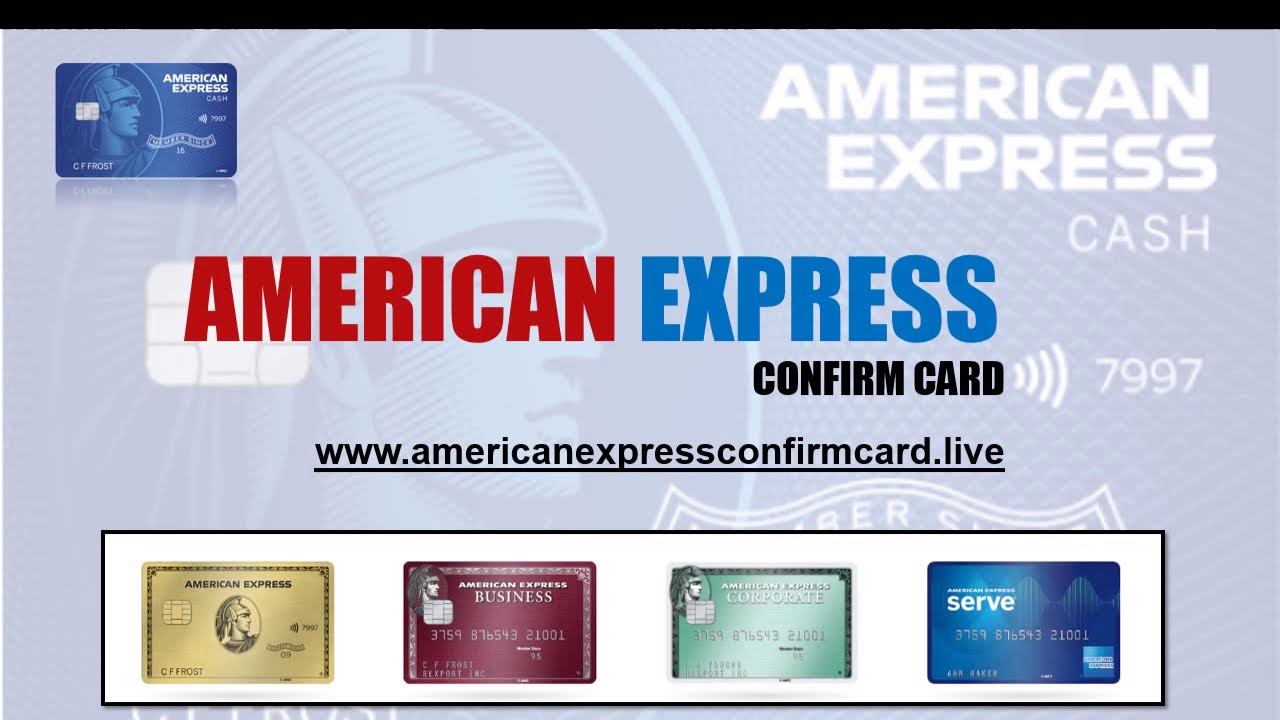A website interface prominently displays "American Express Cash" in the upper left-hand corner, alongside an image of a credit card labeled "American Express Cash," issued to CF Frost, a cardholder since 2016. Directly across on the upper right-hand side, the text "American Express Cash" is mirrored. A large banner below these elements features "American Express," followed by a prompt to "Confirm Card" and a URL: www.americanexpressconfirmcard.live. 

Beneath this section, the images of four distinct types of American Express cards are showcased. The first card appears to be a classic American Express card, the second is an American Express business card, the third is an American Express corporate card, and the fourth is an American Express Serve card. Each card is labeled with the respective cardholder names: CF Frost for the classic card, CF Frost again for the business card, Jaeger for the corporate card, and Ann Baker for the Serve card. All these elements are set against a background that emulates the design and style of an American Express card.